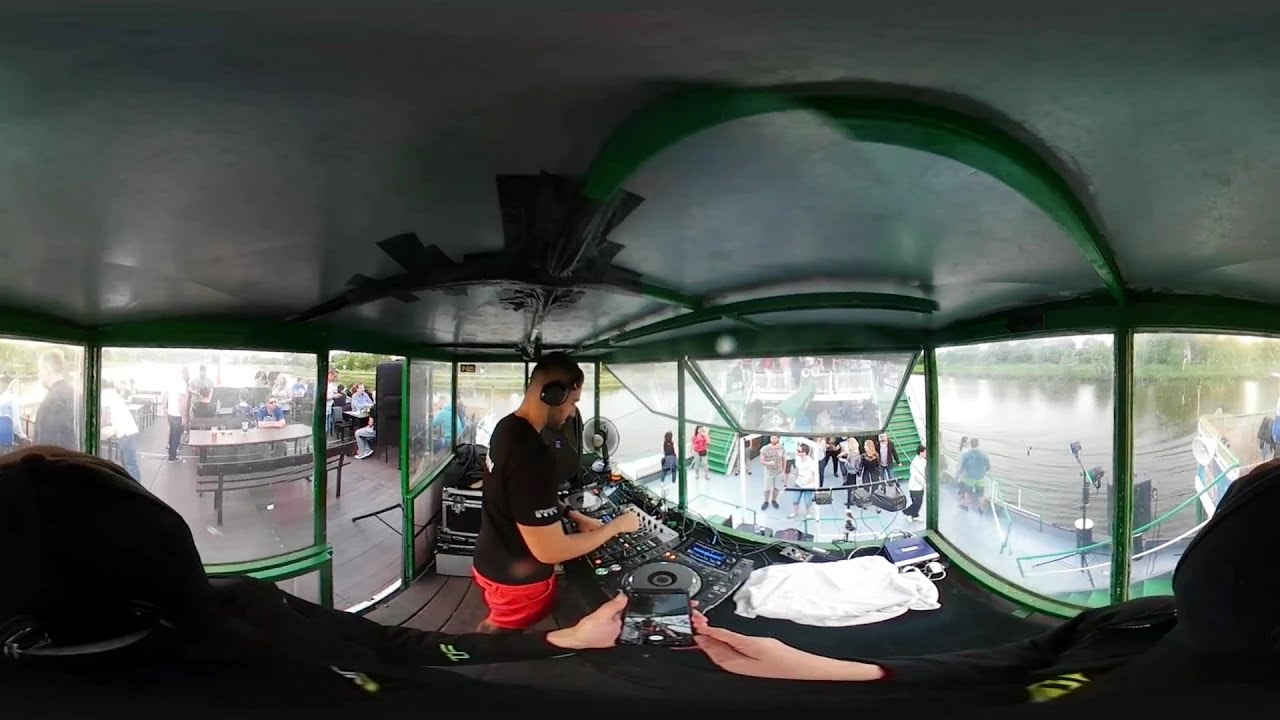This color photograph features a DJ standing in a booth with distinctive green window frames and a silver ceiling. The DJ, who is wearing black headphones, a black short-sleeve t-shirt with unreadable white letters, and red shorts or trunks, is working on an array of electronic equipment including turntables, a CD spinner, and a control dashboard with numerous knobs and screens displaying blue hues. The booth appears distorted due to the lens effect, making it difficult to discern its exact dimensions. In the foreground, there's a visible hand and a white bag on the lower right, while a black cat is visible in the lower left corner. Also visible is a person in black clothing with yellow and green logos on it, looking down at their cell phone. The scene outside the booth includes people milling about, light-colored clothing visible among the crowd, and what appears to be brown tables and benches, possibly in an outdoor area overlooking water. There are green staircases and a deck, suggesting the setting might be near a riverfront or lake, or even on a large boat. The outdoor environment around the DJ's booth adds a dynamic and varied atmosphere to the image.